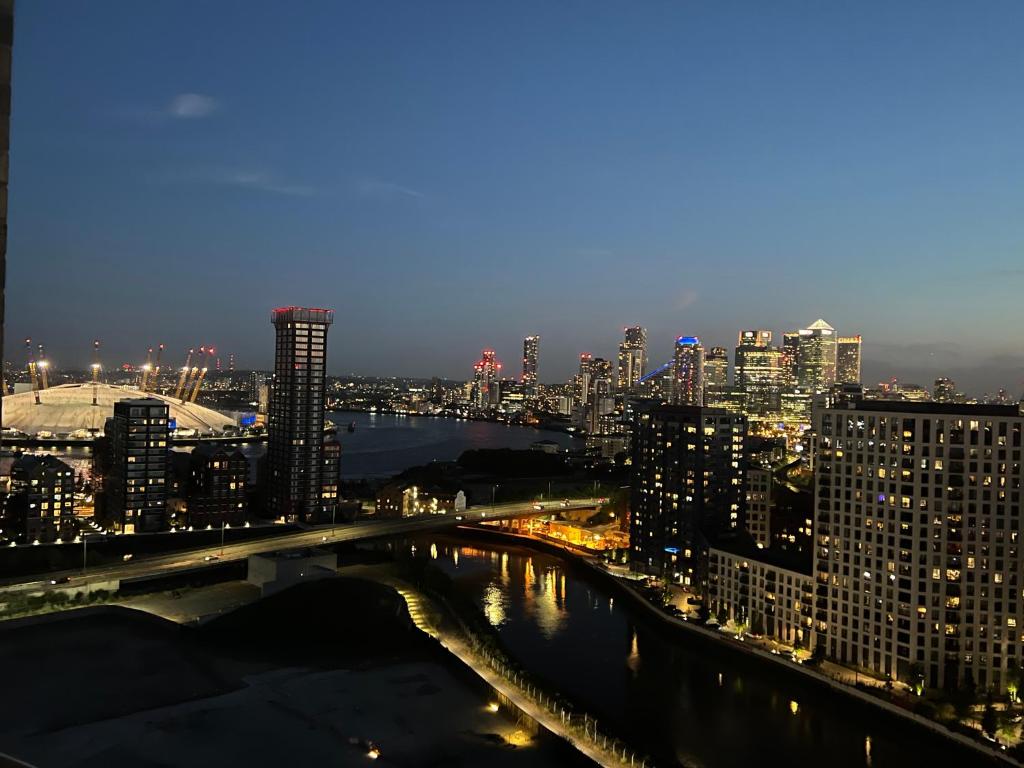Captured at dusk, this aerial photograph showcases a sprawling cityscape encased by dark blue waters. The sky retains a faint blue hue, complemented by myriad city lights in orange, blue, pink, and white. Dominating the left-hand side is a well-lit domed stadium, likely the Superdome, emanating bright white light. The city's landscape is peppered with tall skyscrapers, endlessly stretching into the horizon, where even more buildings are faintly visible. The serene waters reflect the vibrant city lights, accentuating the urban elegance. A prominent pier extends through the water, and multiple bridges, bustling with cars, connect the various parts of the city, hinting at its nautical essence. Roads meander through the metropolis, with a notable highway visible in the distance. The gentle glow of the evening light blends harmoniously with the artificial brilliance, painting a vivid picture of a city transitioning from day to night.